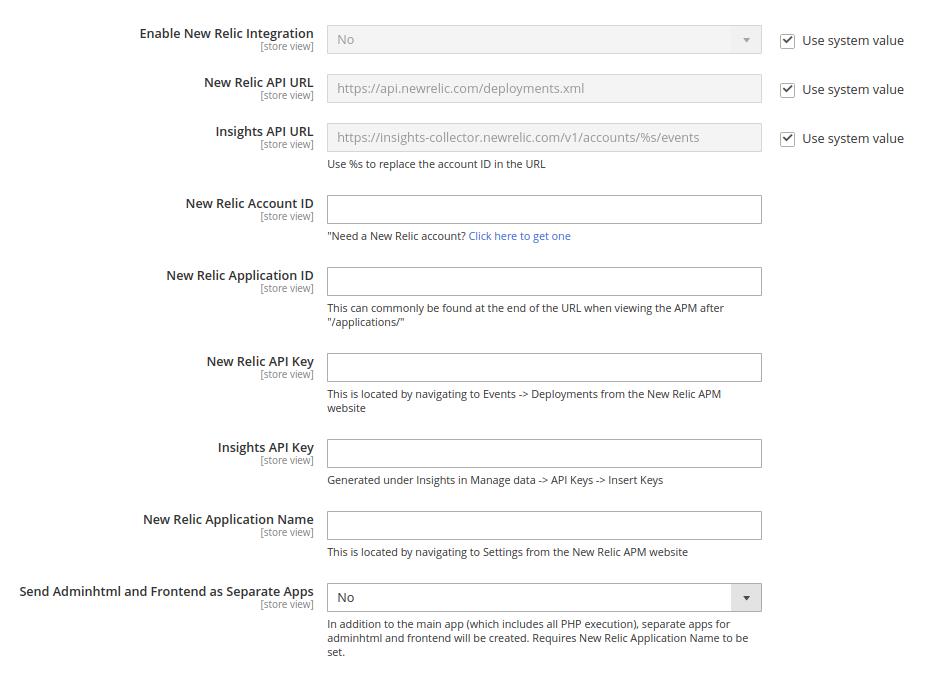A detailed screenshot of a configuration interface for integrating New Relic with a store view. On the left side, a list of configuration options descends vertically, including:

- "Enable New Relic Integration, Store View"
- "New Relic API URL, Store View"
- "Insights API URL, Store View"
- "New Relic Account ID, Store View"
- "New Relic Application ID, Store View"
- "New Relic API Key, Store View"
- "Insights API Key, Store View"
- "New Relic Application Name, Store View"
- "Send Admin HTML and Front End as Separate App, Store View"

To the right of each textual instruction, corresponding input boxes align horizontally. The first box is a toggle switch that currently indicates "No." The following boxes display URLs and input fields, some containing example texts:

1. **New Relic API URL**: `https://api.newrelic.com/deployments.xml`
2. **Insights API URL**: `https://insights-collector.newrelic.com/v1/account/%S/events` with a note saying to replace `%S` with the account ID.
3. **New Relic Account ID**: (Blank input box, with a note below stating to click a link to get one if needed)
4. **New Relic Application ID**: (Blank, with instructions to find this ID in the URL of the APM dashboard)
5. **New Relic API Key**: (Blank, with instructions to navigate to the New Relic APM website, go to events, deployments)
6. **Insights API Key**: (Blank, with guidance indicating this key is generated under Insights -> Manage Data -> API Keys -> Insert Keys)
7. **New Relic Application Name**: (Blank, with a note that this is set via New Relic APM settings)
8. **Send Admin HTML and Front End as Separate App**: Another toggle, currently set to "No," with an additional note clarifying that apart from the main app, which includes all PHP executions, separate apps for administrative HTML and front end will be created if the New Relic Application Name is set.

Overall, the interface appears systematically arranged, accommodating detailed instructions and input fields necessary for enabling and configuring New Relic integration into the store view.